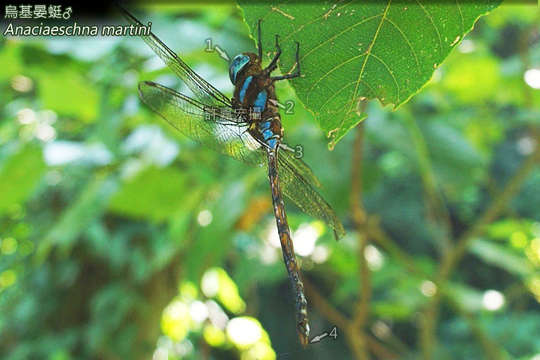In this outdoor photograph, we see a dragonfly perched on a leaf within a backdrop filled with blurred green foliage. The dragonfly features striking blue and black stripes, and the photo has been annotated with numbers to highlight different parts of its anatomy: '1' points to the head, '2' to the body, '3' just above the tail, and '4' at the end of the tail. The leaf it's resting on has a corner nibbled away. Additionally, there is white text in the upper left-hand corner written in what appears to be Chinese or Japanese characters. Below this text, the scientific name "Anna Kryanshia Martini" is shared. The dragonfly's long, transparent wings and three visible legs grasping the leaf add to the intricate details of this snapshot.